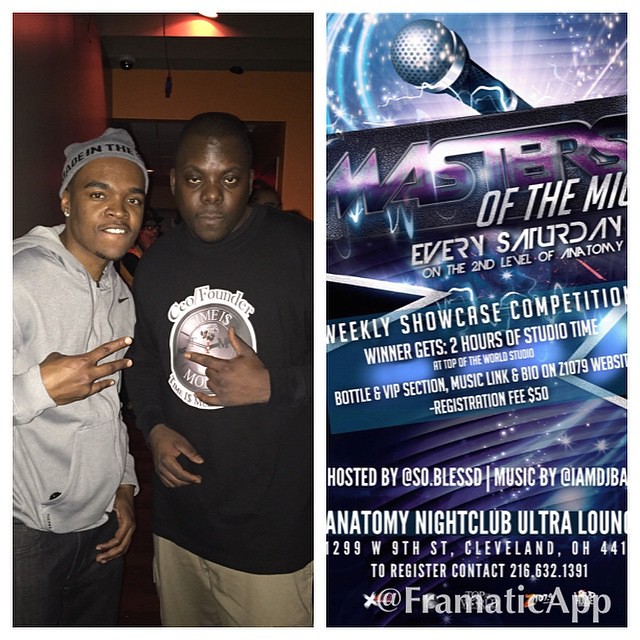The provided image is divided into two distinct, vertically oriented sections. On the left, there is a photograph of two black men posing seriously for the camera. The man on the left is younger, in his 20s, and wears a grey hoodie along with a grey beanie that has black letters. The other man is slightly older, perhaps in his late 20s to early 30s, and wears a black hoodie featuring a white graphic that reads "CEO/Founder. Time is Money." Both men are making hand gestures; the younger man is holding up three fingers while the older man displays the "I love rock" sign.

The image on the right is a partially cropped flyer for an event at Anatomy Nightclub Ultra Lounge, located on West Ninth Street, Cleveland, Ohio. The flyer announces the "Masters of the Mic" event held every Saturday on the club's second level. This weekly showcase competition offers the winner two hours of studio time at the Top of the World Studio, along with a VIP section and bottle service. Additional details include a registration fee of $50, music links on the Z107.9 website, and contact information for registration at 216-632-1391. The flyer also mentions the hosts, "@so.blessed," and the DJ, "@iamdjba." A logo watermark at the bottom right corner reads "@phramaticapp."